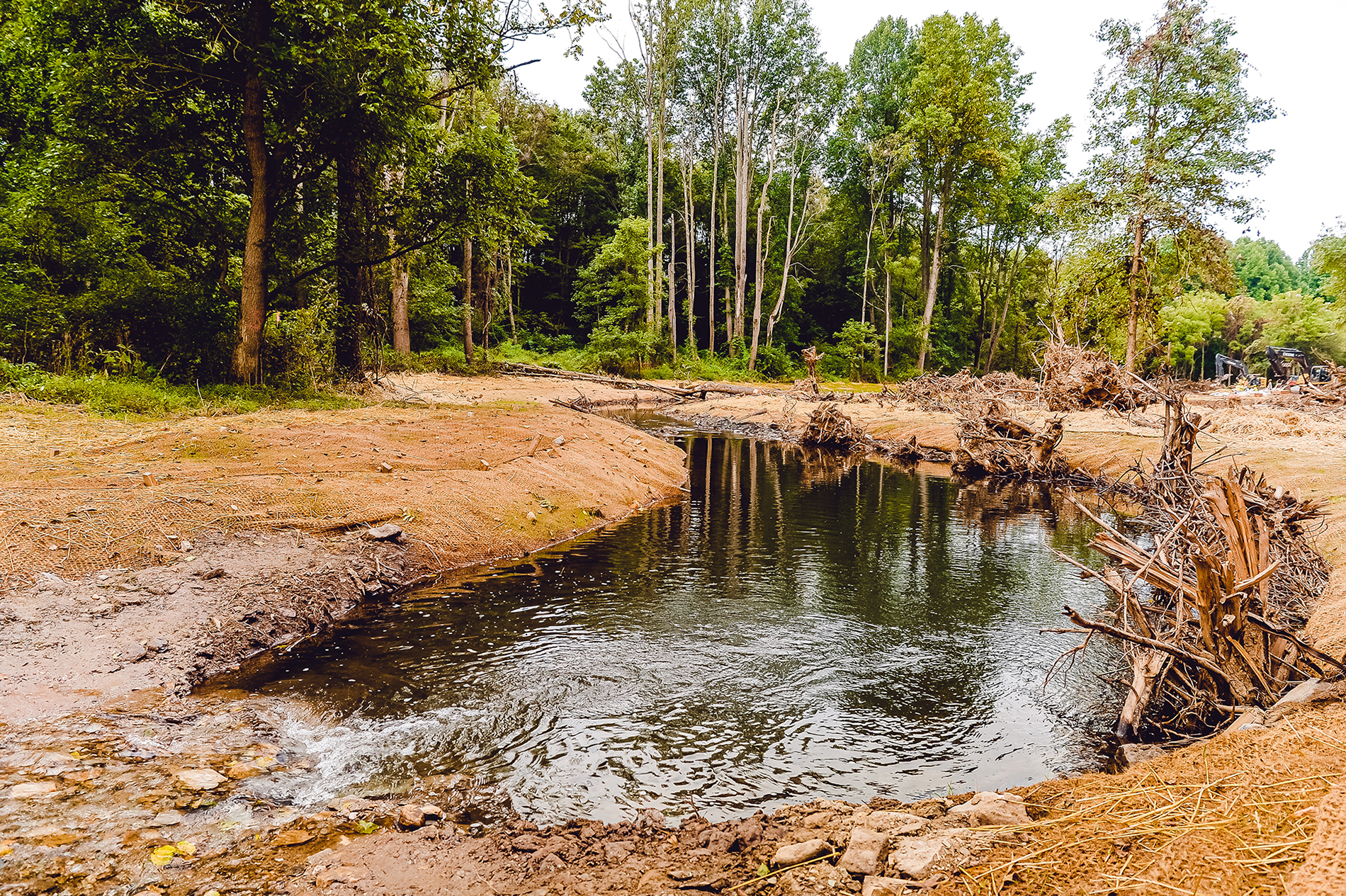The image features a serene creek bordered by tan sandy dirt, trailing off into a small pond that snakes to the right before disappearing from view. Along the banks, several meticulously constructed beaver lodges composed of mud and sticks can be seen, giving evidence of beaver activity. The water itself has a deep green hue and is calm enough to reflect the lush surroundings. 

A dense forest of vibrant, green-leafed trees, including oak, maple, alders, and some coniferous varieties, encircles the creek and pond, forming a picturesque backdrop. Among the foliage, a prominent overturned tree with its roots exposed adds a rugged touch to the natural scene. Scattered around the water's edge are logs and branches, suggesting past logging activities. The overall impression is one of tranquil wilderness, bustling with natural life and activity.